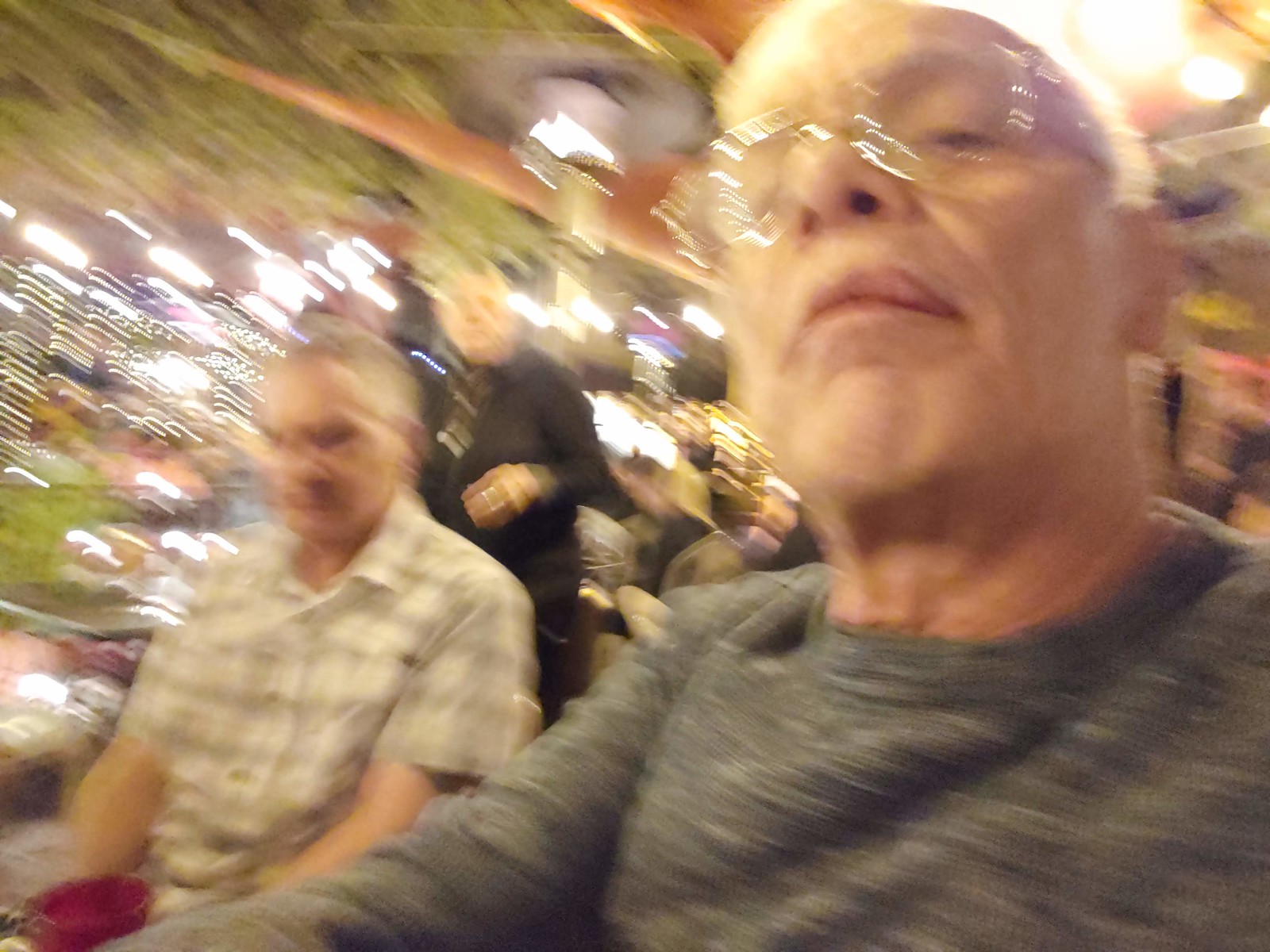The photograph captures a candid, motion-blurred selfie of an older white gentleman wearing glasses and a gray sweatshirt with subtle white patterns. The selfie is taken from a low angle, resulting in an unflattering view up the man's nose. The main subject, positioned on the right side of the frame, gazes downward at the camera. 

To his right stands another older white individual dressed in a short-sleeved, white and gray flannel button-up shirt. A third older white person, slightly obscured and blurred in the background, appears to be donning a black suit with a black tie. The setting hints at a restaurant ambiance, indicated by several out-of-focus lights in the backdrop, adding to the image's overall blur and sense of motion.